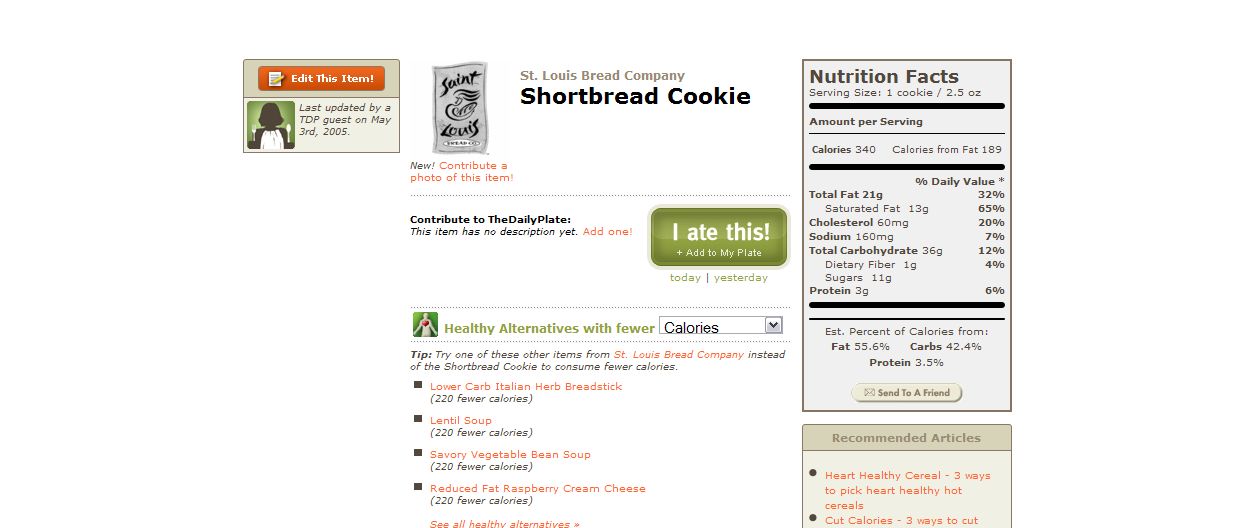This image captures a computer screen displaying a label for a shortbread cookie from the St. Louis Bread Company. Prominently featured in the center of the label is the name of the product, "St. Louis Bread Company Shortbread Cookie," along with a diminutive logo of the St. Louis Bread Company. Below the logo, there is a section dedicated to healthier alternatives, offering options with lower calorie counts. However, the text providing details about these alternatives is somewhat unclear and difficult to read. To the right side of the label, a boxed area presents the nutrition facts for the shortbread cookie, giving consumers detailed information about the cookie's nutritional content. An edit button is visibly positioned to the left of the label, indicating that the image is indeed a screenshot of a computer display where the label might be in the process of being edited or reviewed.